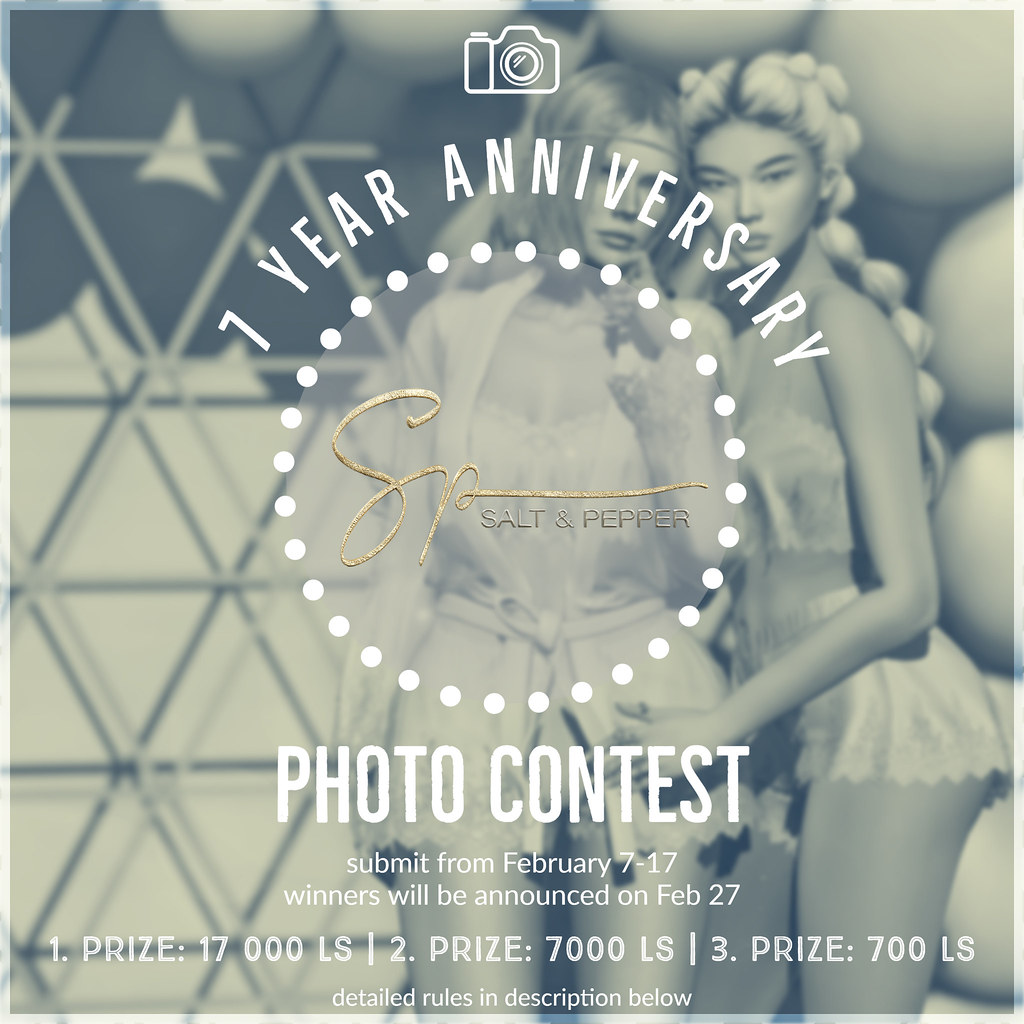This image is a screenshot of an Instagram post commemorating the one-year anniversary of the "Salt-N-Pepper" photo contest. At the top center, there's a clipart-style camera, and below it, "one year anniversary" is written in curved letters. Surrounding the gold-lettered "SP Salt-N-Pepper" logo is a circle made of white dots with a transparent pink inner circle. Below the logo, large white letters announce the "photo contest" and state that submissions will be accepted from February 7th to 17th, with winners announced on February 27th. Detailed rules are mentioned to be in the description below. The prizes are listed as follows: first prize is 17,000 LS, second prize is 7,000 LS, and third prize is 700 LS. In the background, a blurry black-and-white image features two women, possibly 3D-rendered models, wearing lingerie. One woman in the center is slightly tilting to the right, while another woman with braided ponytails stands to the right, hugging her. The image is stylized to emphasize the theme of a beauty contest.